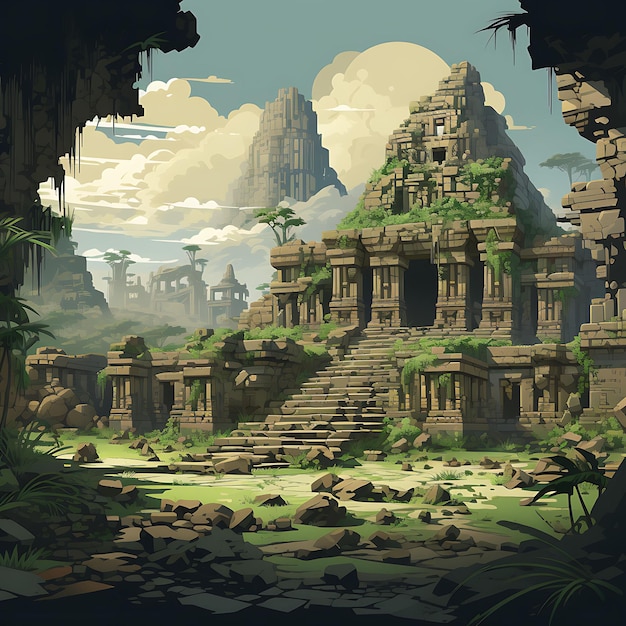This image is a digital illustration depicting the serene yet mysterious ruins of ancient temples, rendered in a detailed and colorful cartoon style reminiscent of a children's video game or animated show. The dominant colors are green and brown, with lush vegetation consisting of green moss creeping over the crumbling rocky pillars and staircases. The main focus is a large, light brown temple, centered slightly towards the right side of the scene. This temple features a grand staircase with approximately twenty steps ascending to two levels, culminating in a conical peak.

To the left, peeking out from the overcast greenish-blue sky with a faint moon obscured by clouds, is another ruin subtly hidden among the clouds. The backdrop includes more temples, enhancing the ancient and mystical atmosphere of the artwork. The ground in the foreground and the curved, crumbling structures on both sides emphasize the aged and deteriorated state of these magnificent historic sites, inviting viewers to imagine the grandeur they once held.